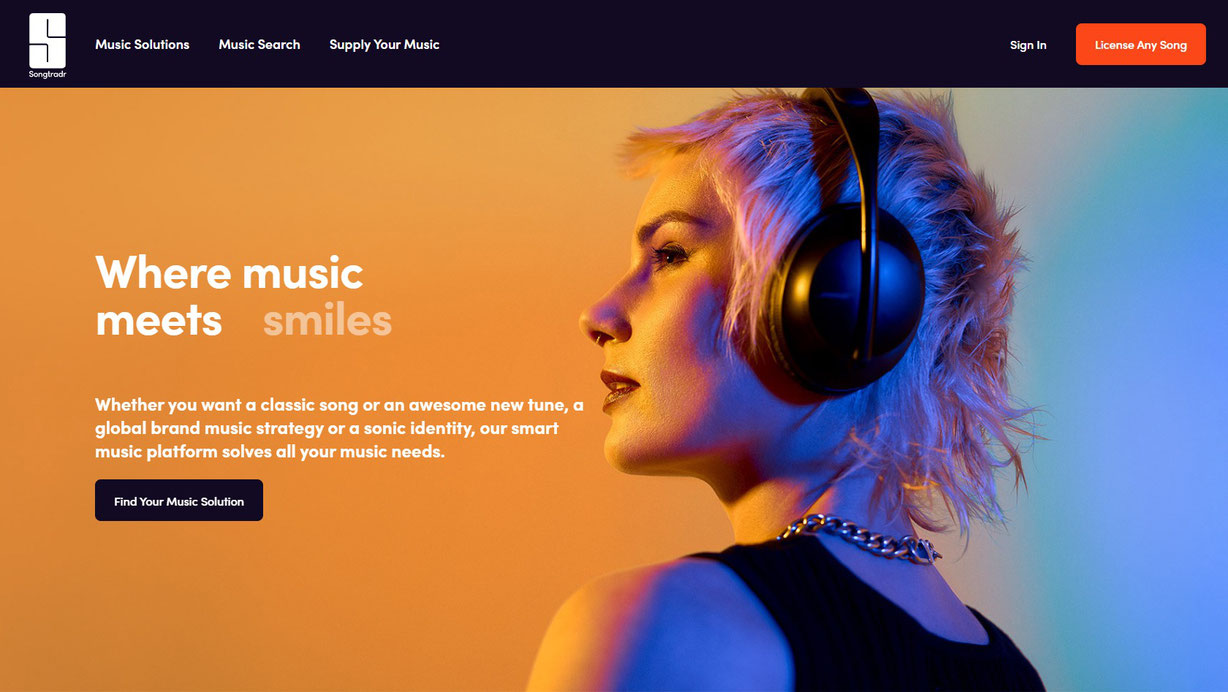This screenshot of a website captures the homepage of Songtradr, a music licensing platform. At the top, a black rectangular banner spans the width of the page, featuring an icon with a large, capitalized 'S' and the brand name 'Songtradr' written in white, sans the letter 'e', making it 'S-O-N-G-T-R-A-D-R'. To its right, text reads "Music Solutions, Music Search, Supply Your Music."

Across the top, there's a navigation menu including options for user sign-in and a prominent red button labeled "License Any Song." Below this section, an image features a woman wearing headphones and a chain necklace, dressed in a sleeveless black top. She has noticeable eye makeup and lipstick, with short hair that appears blond with slight pink highlights. She gazes to the left of the frame. 

Overlaying this image, text reads, "Where Music Meets Smiles." Below, additional text states, "Whether you want a classic song or an awesome new tune, a global brand music strategy, or a sonic identity, our smart music platform solves all of your music needs." A black button below this invitation encourages visitors to "Find Your Music Solution."